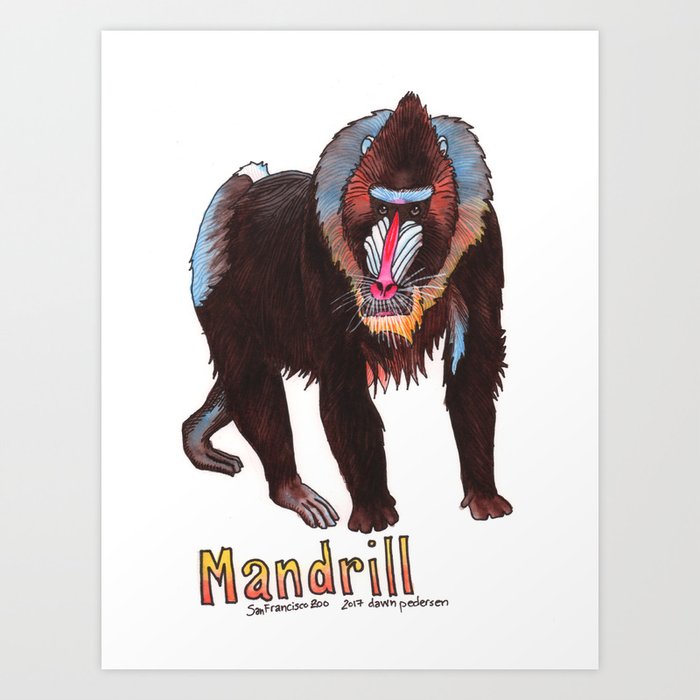This is a detailed illustration of a mandrill, set on a white rectangular piece of paper with a beige background that has a light gray edge, thicker on the sides and thinner at the top and bottom. The illustration prominently features a mandrill, an animal closely related to baboons, standing on all fours with its knuckles down and facing towards the right while looking towards the viewer. 

The mandrill has a striking red nose with a white striped design running up towards its forehead, accented by piercing eyes and noticeable whiskers. Above its eyes, the mandrill seems to have a blue eyebrow-like feature, while the snout below the nose is white. Its fur is predominantly dark brown with a mane around its head that displays a blend of blue on top and shades of brown, red, and orange below. Additionally, blue accent fur can be observed on its legs and inner arms, with blue also present on its butt and hints of red on its belly.

Wrapping up this intricate illustration are textual annotations at the bottom of the paper, which read: “Mandrill,” boldly outlined in yellow, orange, and red colors, and “San Francisco Zoo 2017” followed by the name “Dawn Henderson” in smaller black text.